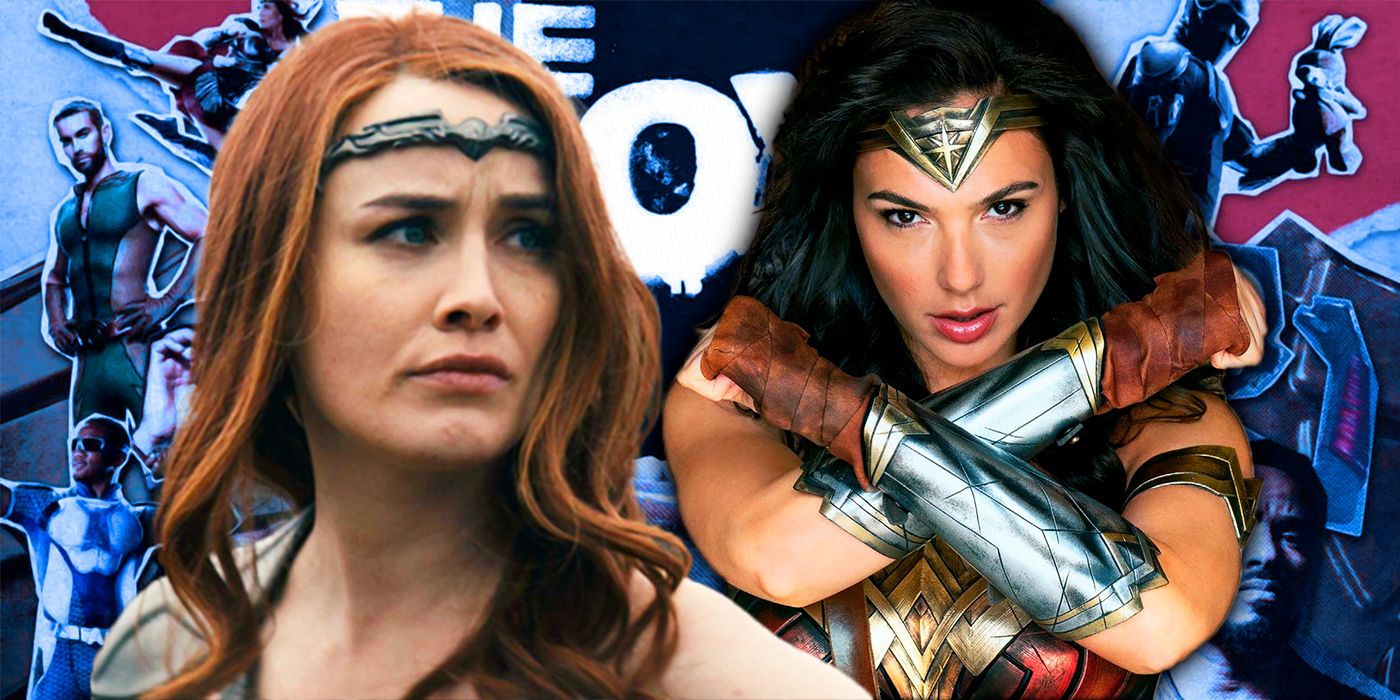The image features two women who resemble superheroes. The woman on the left has long red hair and is wearing a silver headband, looking over her left shoulder. The woman on the right has long black hair, adorned with a gold headband. She is wearing brown leather gloves, a silver gauntlet across her forearms, and a reddish-goldish top. She has her arms crossed and is sporting red lipstick. Both women appear to be standing in front of a wall covered with drawings of various superheroes. Among the sketches, there are male superheroes, a blue and white ranger-like figure, a green superhero, and a woman in mid-kick. The background, possibly a poster, is vibrant with colors like red, blue, and pink, featuring characters in fighting attire, helmets, and armor.